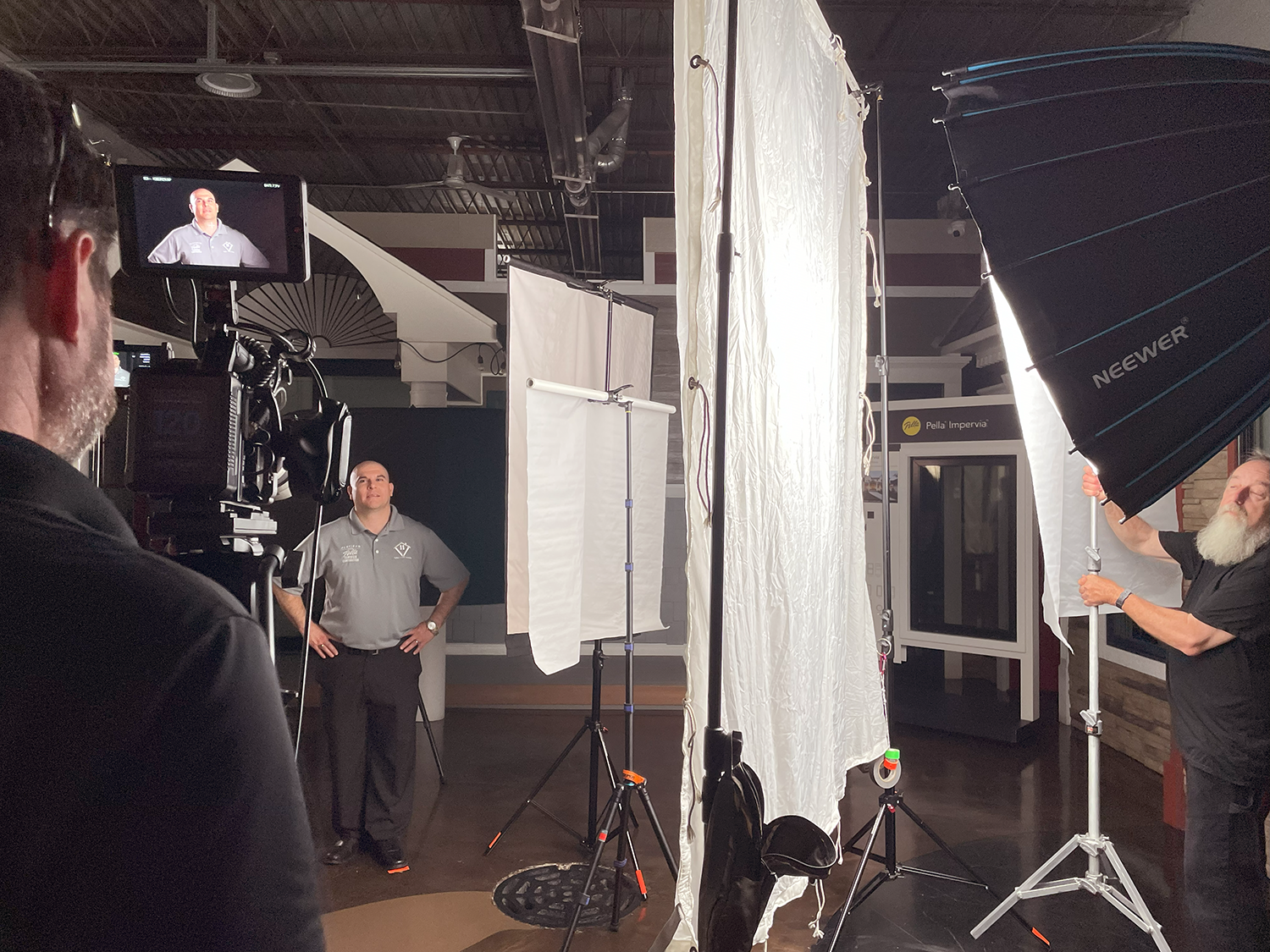In the photo, set in a professional studio with a black ceiling, a bald man wearing a gray polo shirt adorned with logos and black pants stands poised for an interview or commercial shoot. He is surrounded by various lighting fixtures, including a prominent large white curtain in the center and several smaller white screens. In front of him, a man with a white beard dressed in black is adjusting a lighting fixture, while another man wearing a black shirt operates a camera aimed at the bald man. The scene also includes a small monitor displaying the focused subject, further emphasizing the detailed setup typical of a small family business or company filming environment.